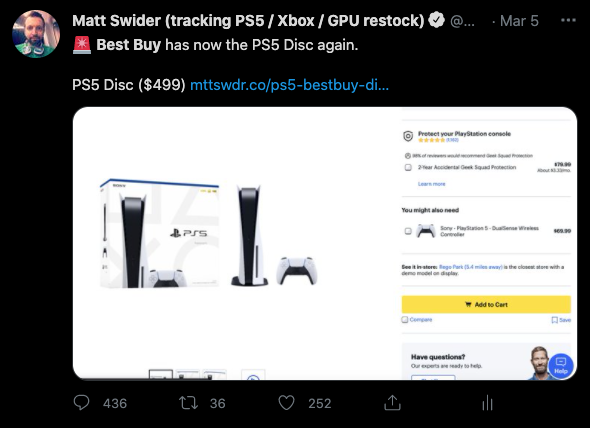The image showcases the interface of a Twitter or X page with a dark background. In the top left corner, there is a profile picture of a man looking directly into the camera, identified as Matt Sweider. His profile description reads, "Tracking PS5/Xbox/GPU restock." A verified checkmark confirms the authenticity of his account. The timestamp indicates the post was made on March 5, and the content announces that Best Buy now has the PS5 disc version available for $499, including a web link for more information.

Beneath this tweet, displayed against a white background, is detailed product information. To the left, there's an image of a PlayStation 5 console. On the right, text suggests options to "Protect Your PlayStation Console," with a two-year protection plan available for $79.99, though this option is not selected.

Further down, the page mentions additional accessories, such as a "Sony PlayStation 5 wireless controller," which is pictured in its box and marked at $69.99. This option is also not selected. The text repeats the controller's price as $69.99, emphasizing accessibility to view it in-store, followed by some blurred text. There is a prominent "Add to Cart" button.

In the bottom right corner, there's a customer service prompt stating, "Have questions? Our experts are here to help," with an accompanying help button. Additionally, at the very bottom of the interface, social interaction icons include a speech bubble with "436" next to it, an up arrow with "36," a heart with "252," and another up arrow, indicating various user interactions such as comments, likes, and upvotes.